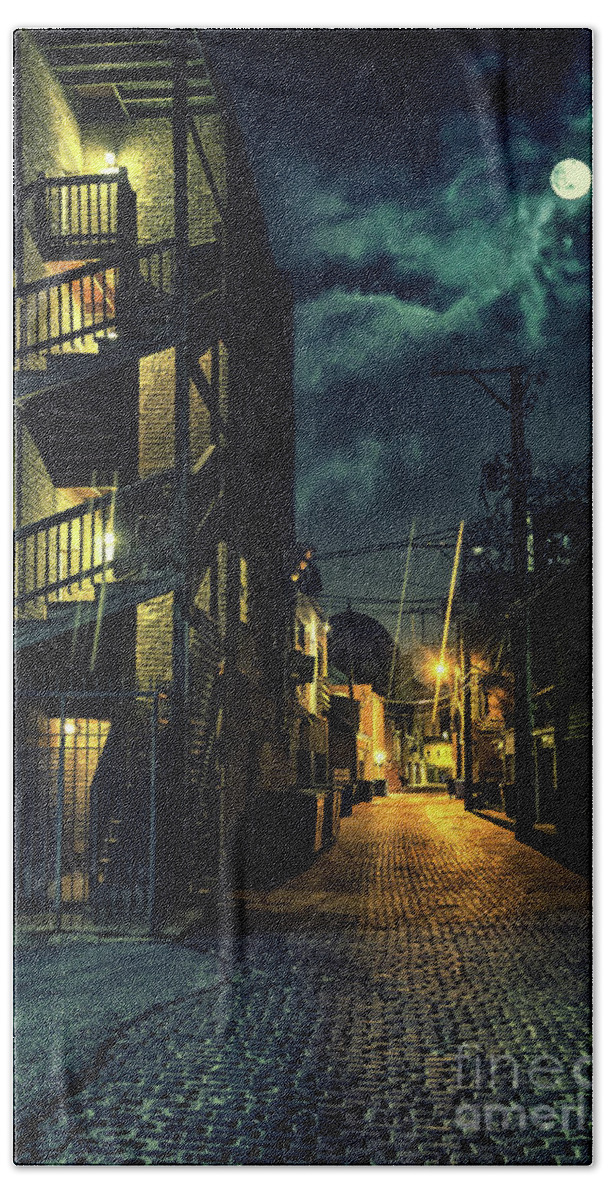The image is a vertical, moody night scene in an urban setting that captures the nostalgic ambiance reminiscent of a 1930s detective novel cover or an album cover like Ziggy Stardust. The sky is cloudy with a prominent full moon casting a dim light on the scene below. A cobblestone street stretches through the lower part of the image, guiding the eye into a dimly lit back alleyway. On the left-hand side, a three to four-story brick apartment building, featuring wooden fire escapes, dominates the scene, illuminated by either street lights or the moonlight, which casts a yellowish glow across the scene. The poorly lit buildings and the sporadic street lights add to the overall somber and mysterious atmosphere. Telephone poles and a faint human figure in the distance add to the urban decay, while a white watermark in the bottom right hints at an artist's signature or title, possibly "something omen" or "American."